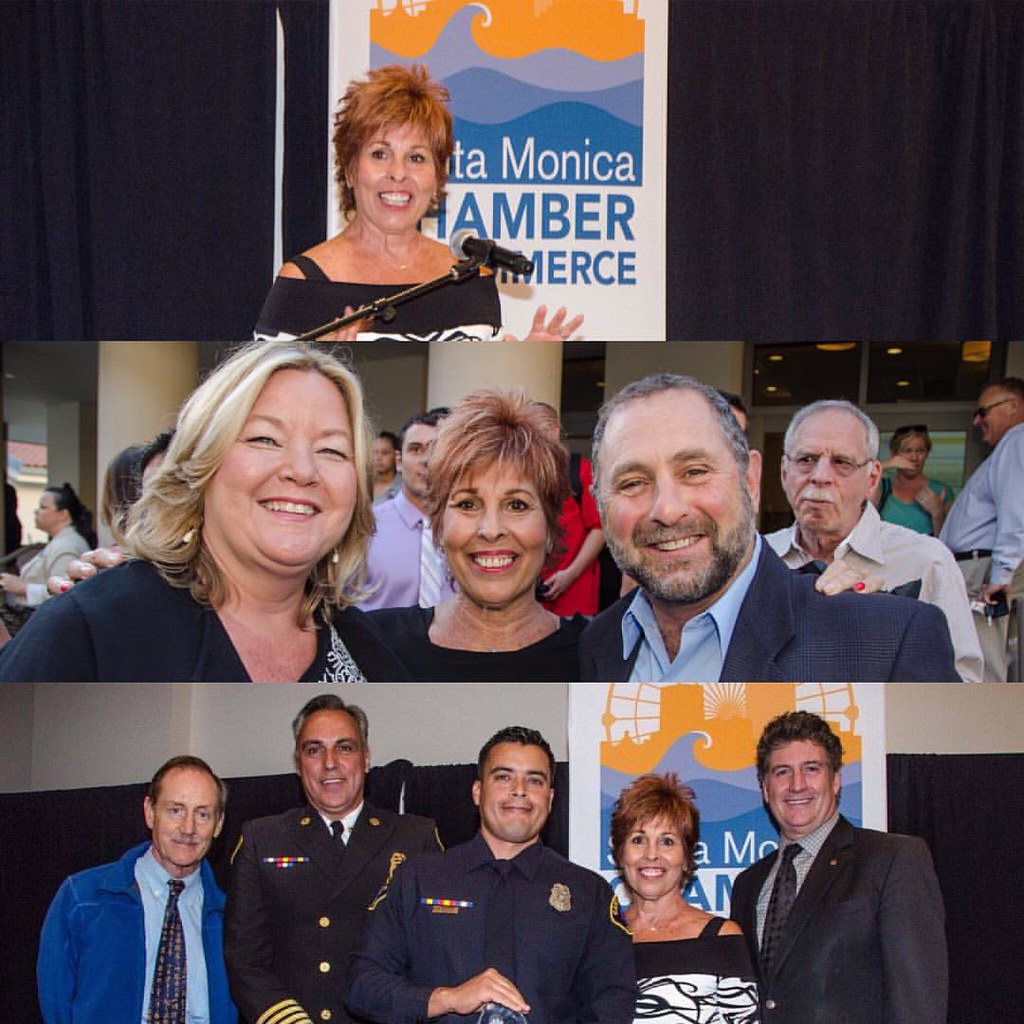The composite image consists of three horizontally arranged photographs. In the top photograph, a woman with short, spiky red hair stands behind a microphone, smiling and gesturing with both hands. She is wearing an exposed-shoulders top featuring navy blue straps and a white lower section. The backdrop is a dark blue curtain with a "Santa Monica Chamber of Commerce" poster prominently displayed, depicting an orange sky and blue ocean waves. The middle photograph captures three individuals posing together. The woman from the first photograph is in the center, flanked by a smiling blonde woman on her left, dressed in a dark blue top with white embellishments, and a bearded man with short brown and gray hair on her right, wearing a blue shirt and dark blazer. A crowd is visible in the background. The bottom photograph shows five individuals posing for a group photo. From left to right: an older man with male pattern baldness and a mustache, wearing a blue jacket, light blue shirt, and tie; a smiling man in a military uniform with short grayish hair; a man in a law enforcement uniform with short black hair, possibly Hispanic; the same woman from the earlier photographs; and finally, a smiling man with curly dark hair, dressed in a dark suit and a white and blue checkered shirt with a dark tie. They stand in front of the same "Santa Monica Chamber of Commerce" poster as in the top photograph, which is attached to a wall that is white on the upper half and black on the lower half.